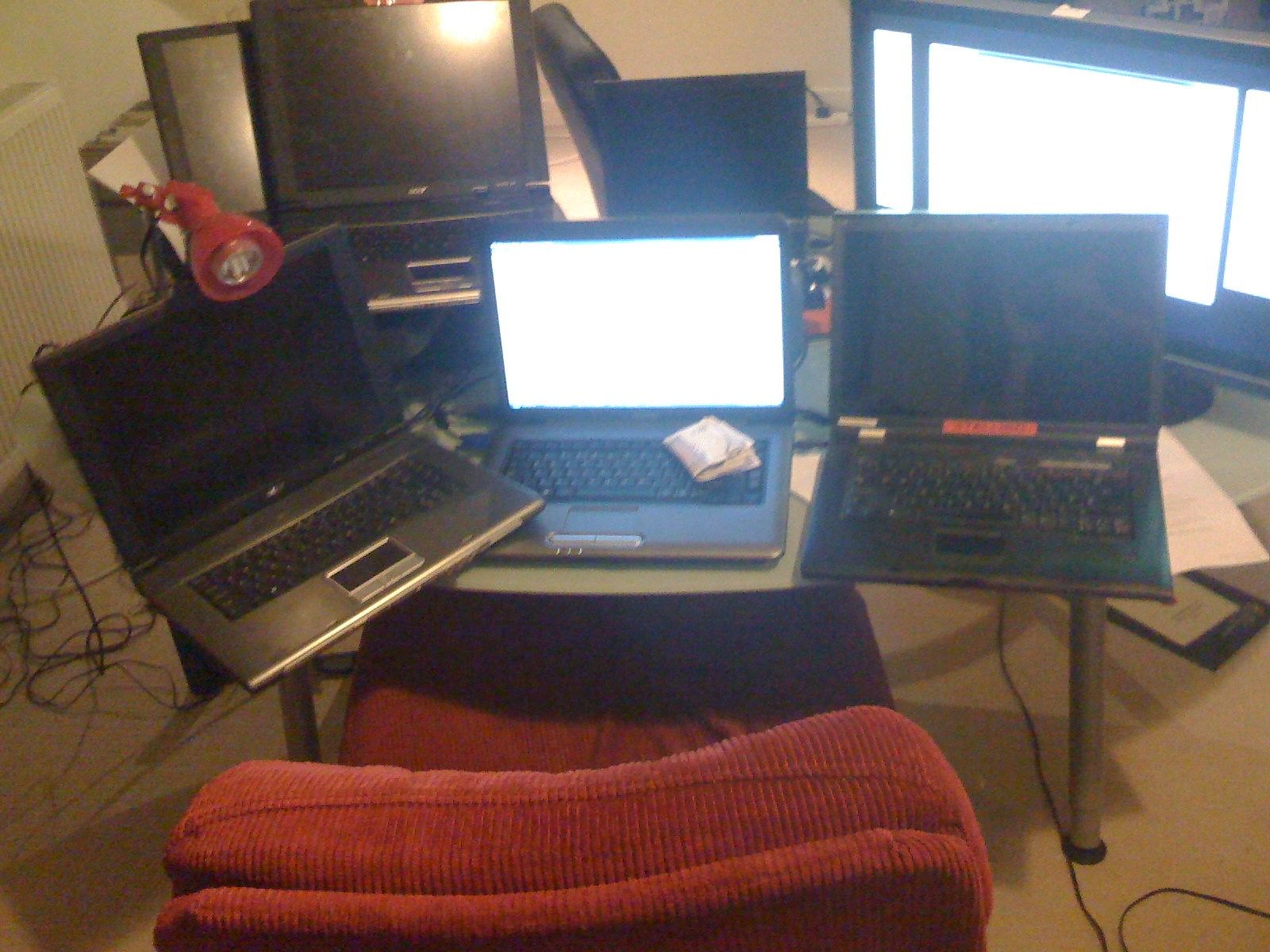This photograph depicts a well-used computer setup, likely in a basement or a hobbyist's workspace, possibly a computer repair shop. Dominating the foreground is a plush, red velvet chair that resembles a recliner. Overlapping the chair is a two-tiered computer table that holds three laptops with their screens open. The central laptop's screen is illuminated, displaying a white screen, while the laptops on either side are turned off and have dark screens. A red desk lamp is clipped above the central laptop, casting a glow over the setup.

In the background, additional computers—around five or six—are stacked, some of which have their screens facing the chair. The room is dimly lit, with reflections of an overhead light visible on one of the laptop screens. The floor is covered with grey carpet, and numerous black power cords snake underneath the desk, adding to the chaotic ambiance of the space. The overall scene suggests a cluttered, yet functional area dedicated to working on or repairing older, non-widescreen laptops.